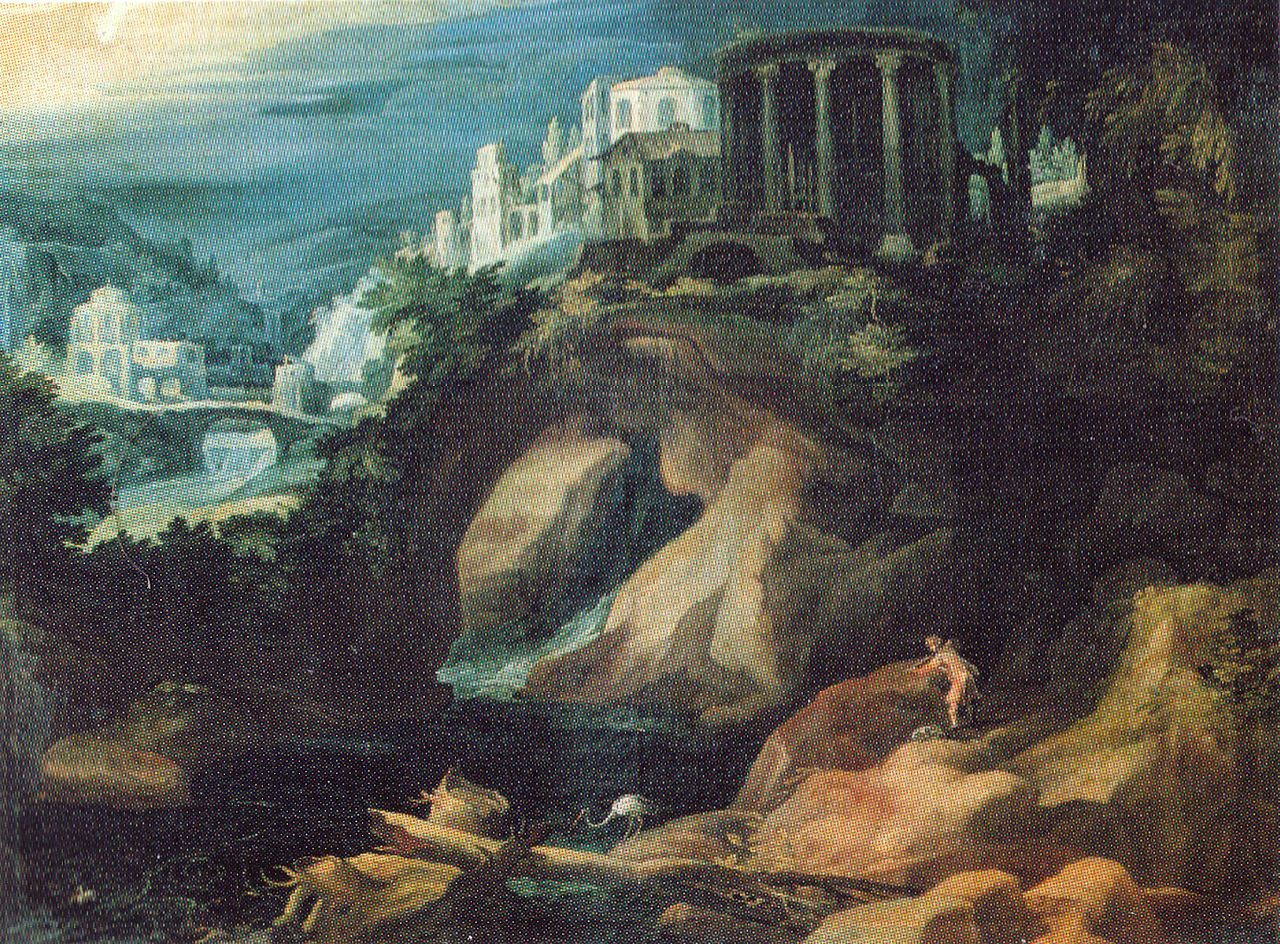This painting depicts an ancient cityscape on a hill, next to a rocky embankment leading into a river or lagoon. The lower part of the image is dominated by a landscape of large boulders and rocks, with some greenery such as trees and bushes. In the bottom right corner, a small figure of a man can be seen, seemingly eyeing a white bird, possibly a seagull or a crane, with an orange beak and long neck, which is feeding in the water. Above the embankment, a series of white buildings, hinting at an old city, are situated atop the hill. To the right, there's a waterfall or large rock structure spilling into the water. The sky is filled with clouds, and the overall color palette includes shades of yellow, white, blue, gray, green, and tan. The painting, likely created by hand in either oil or watercolor, offers a detailed and atmospheric representation of a serene yet rugged landscape, highlighted by the interaction between the solitary figure and the bird.